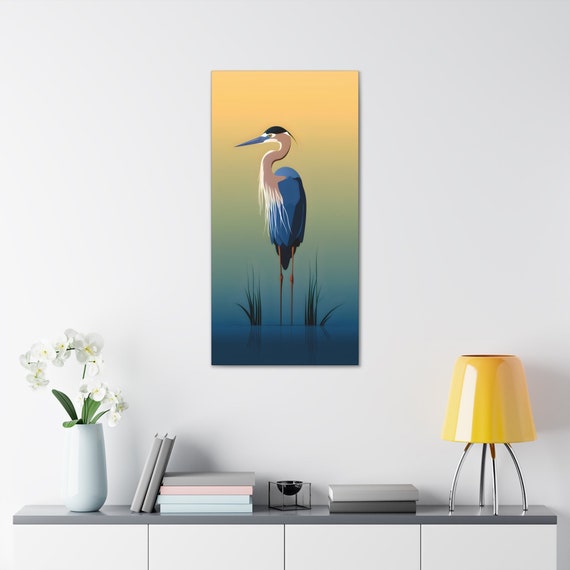This indoor photograph, likely a stock image with an edited painting, captures a neatly arranged scene reminiscent of a living room or office. Central to the image is a vertically oriented painting of a serene heron, showcasing its blue feathers, black tail feathers, and a distinctive S-shaped white neck. The heron's black-capped head and blue beak are turned left, standing gracefully in blue water with tufts of green grass at its feet. The painting's ombre background transitions from a golden hue at the top to teal in the middle, fading into blue at the bottom.

This striking artwork hangs on a pristine white wall, directly above a sleek white shelf with a gray tabletop. The shelf hosts an orderly array of books in shades of white, gray, and pink. To the left, a white flower pot holds delicate white flowers, while to the right, a modern yellow desk lamp with four slender silver legs adds a contemporary touch. This meticulous setup focuses on the art print, highlighting its tranquil beauty and the elegance of the overall arrangement.